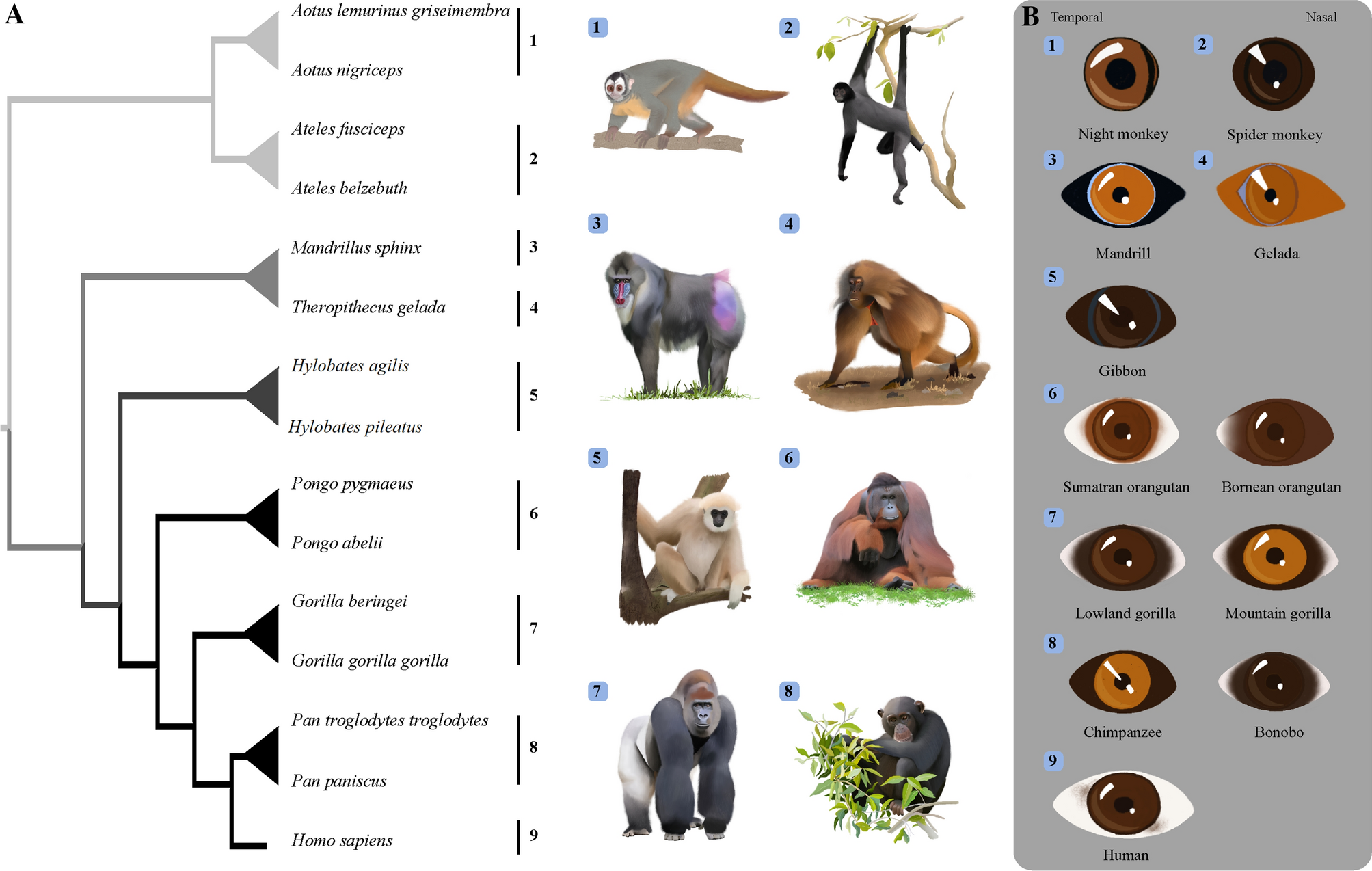The image is a comprehensive and colorful chart focused on various species of primates, including monkeys, gorillas, and lemurs. At the center, it features detailed illustrations of nine different primates, each labeled with both their common and scientific names, arranged from the smallest to the largest species. To the left, the names of the primates are listed vertically, with connecting lines color-coded from light to dark gray, grouping related species. On the right-hand side, there’s a light gray box containing small illustrations depicting the diverse eye shapes and colors of these primates. Most eye colors are variations of brown, reflecting the actual eye colors of the species. This chart includes eye illustrations from species like the night monkey, spider monkey, mandrill, gelada, gibbon, Sumatran orangutan, Bornean orangutan, lowland gorilla, mountain gorilla, chimpanzee, bonobo, and what appears to be a human ("Homo sapiens"). The visual representation is both informative and engaging, offering a rich insight into the physical traits of these fascinating primates.